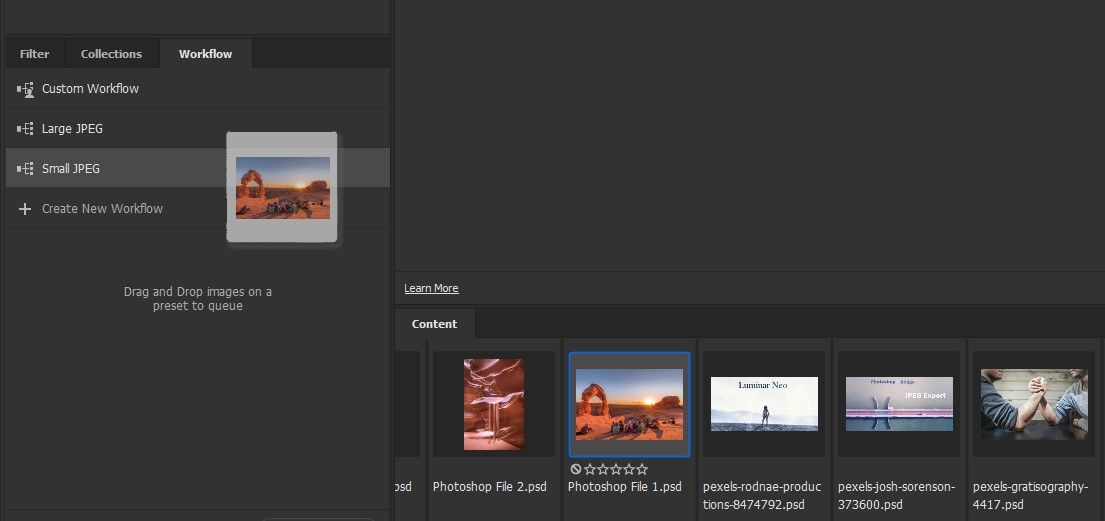Here is a cleaned and detailed caption based on the description:

---

The image captures a screenshot of an online application displayed on a desktop computer, featuring a user interface with a dark gray background. The screen is divided into two sections: a narrower left-hand panel and a larger right-hand panel. 

The left-hand panel contains three tabs lined up at the top, each labeled in white text against a black background. The tabs are, in order: "Filter," "Collections," and "Workflow," with "Workflow" highlighted. Below the tabs, a list of workflow options is displayed. These options include "Custom Workflow," "Large JPEG," and "Small JPEG." Adjacent to these options, on the right side, is a preview image of a landscape scene characterized by a red terrain under a gray sky.

The right-hand panel showcases a larger viewing area, with an upper section that appears empty and a lower section that includes a strip of five thumbnail images. The second thumbnail is highlighted, matching the image displayed in the left-hand panel.

---

This detailed caption clearly describes the visual elements and layout of the screen.